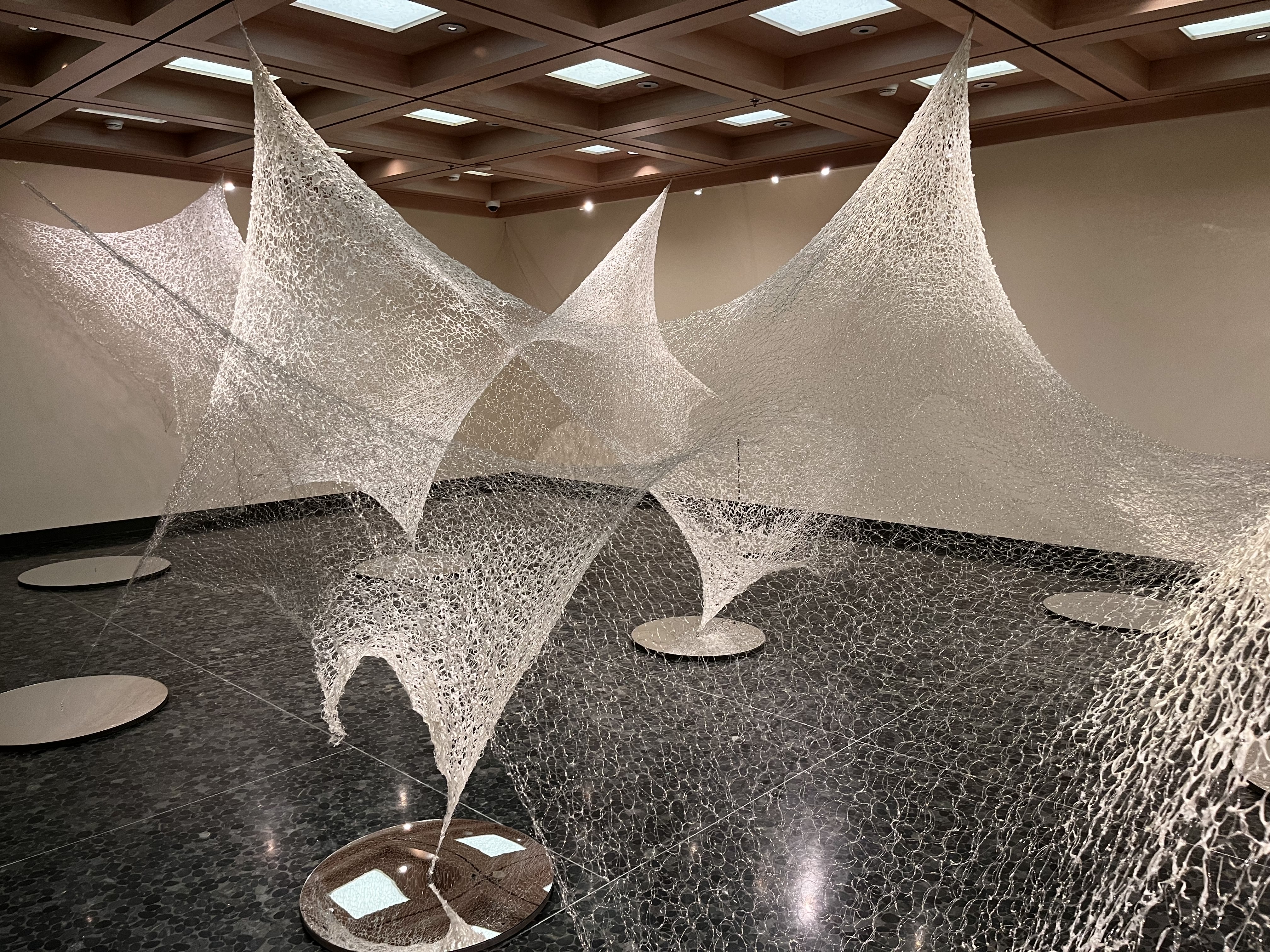The image depicts a large, empty room that appears to be an art installation or museum exhibit. The room features a dark gray or black floor, likely made of marble or linoleum, and light tan or dark beige walls. The ceiling is composed of brown wood with recessed lighting in square sections, contributing to a well-lit environment. The striking centerpiece of the room is a transparent, white fabric sculpture, resembling a massive, intricate spider web or cobweb. This flowing, web-like design is both diaphanous and tensile, creating a futuristic and abstract appearance. The sculpture is anchored to the floor by several circular disks and stretches up to the ceiling where it is secured by hooks. Additional lighting from the floor enhances the delicate, see-through nature of the fabric, making the whole installation appear ethereal and dynamic.